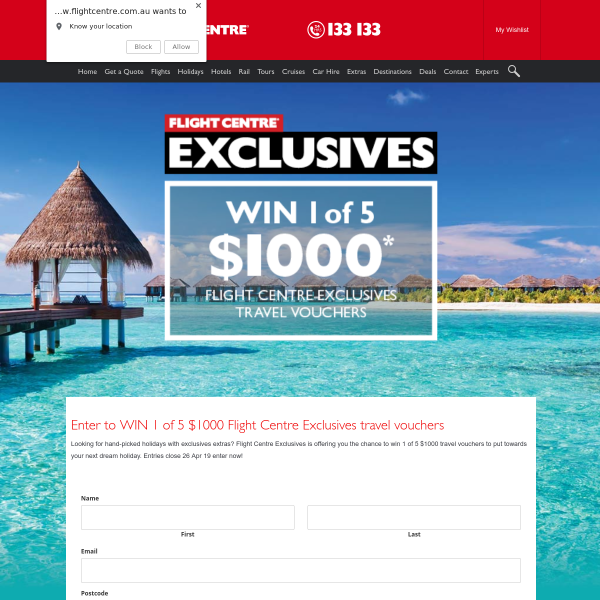This image is from the Flight Centre website and features a stunning tropical scene. The focal point is a serene, turquoise blue expanse of water. A wooden boardwalk extends over the water, leading to a quaint hut positioned at the end. Across the water, the opposite shore is visible, adorned with a sandy beach, lush trees, and several small huts designed for tourists.

The website itself has a distinctive red ribbon across the top with "Flight Centre" displayed in bold white lettering. Adjacent to it is a phone icon accompanied by the number 133133. A location prompt from FlightCenter.com.au is visible, obstructing part of the webpage's header.

Below the image, a black ribbon with the word "Exclusives" in white capital letters is prominently displayed. Further below, a white rectangular box announces a chance to "win one of five $1,000 Flight Centre Exclusive Travel Vouchers." Additionally, there is an entry form requiring your name and email address to participate in the sweepstakes.